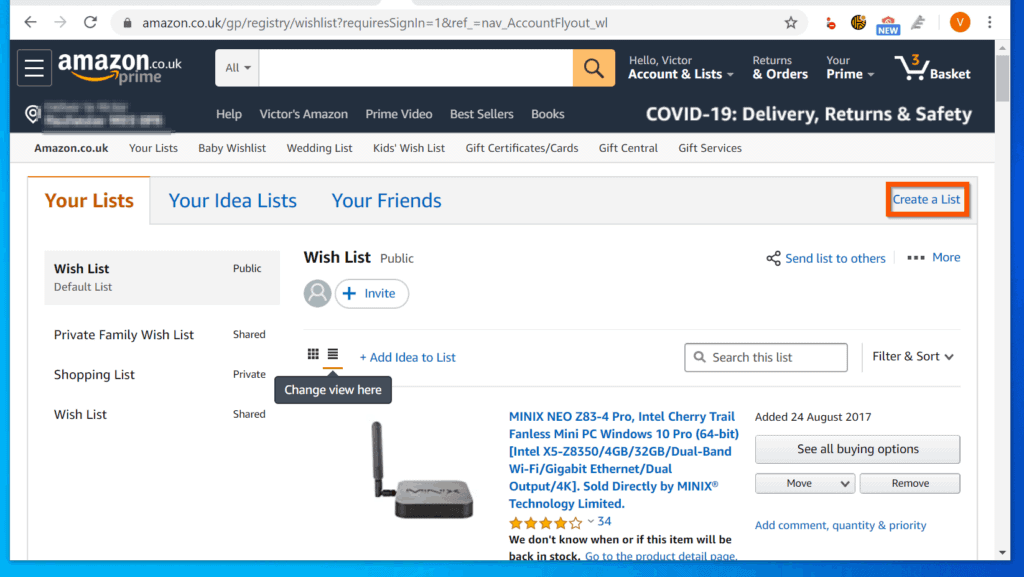The image depicts a user profile on the Amazon.co.uk website, where the user frequently shops. At the top, the URL "amazon.co.uk" is visible, indicating the UK version of Amazon. The page is part of a registry, which serves as a wish list. Although the person's name and location are blurred out, it is identified as "Victor's Amazon."

The layout shows standard navigational options including "Prime Video," "Bestsellers," "Books," and a "Help" icon. There's a search box for entering queries. Victor has three items in his shopping basket, as indicated by the number "3" highlighted within the basket icon. Information related to COVID-19 delivery, returns, and safety is also displayed on the page.

Victor's lists are divided into different categories: his public wish list, a private family wish list that is shared, and a private shopping list. A small icon suggests an option to invite others to view his lists. One specific item on Victor's public wish list is the Minix Neo Z83-4 Pro Intel Cherry Trail fanless mini PC with Windows 10 Pro 64-bit, Ethernet, dual output, and Wi-Fi, sold directly by Minix. This item has a four-star rating based on 34 reviews and was added to his wish list on August 24, 2017. Options available for the item include "See All Buying Options" or removing it from the list.

A prominent red box outlines an option to "Create a List." Additional options for "Your Idealist" and "Your Friends" are written in blue, while "Your List" is highlighted in orange.